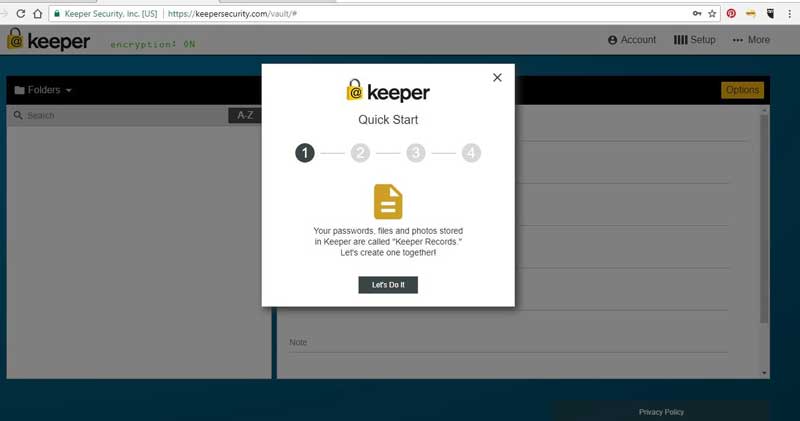**Caption:**  
A screenshot of the Keeper app's onboarding process is displayed. The app appears to be focused on security, given its logo featuring a gold padlock. At the center of the page, a prominent popup stands out, dimming the background. The brightly illuminated popup is labeled "Quick Start" and showcases a step-by-step guide, with the current step being the first one. The text reads: "Your passwords, files, and photos stored in Keeper are called Keeper records. Let's create one together." Below the text is a black button with white text that says "Let's Do It." Above the instructional text sits an icon resembling a yellow variant of the Google Docs logo, featuring two white lines. This image captures the initial stage of securing files within the app.